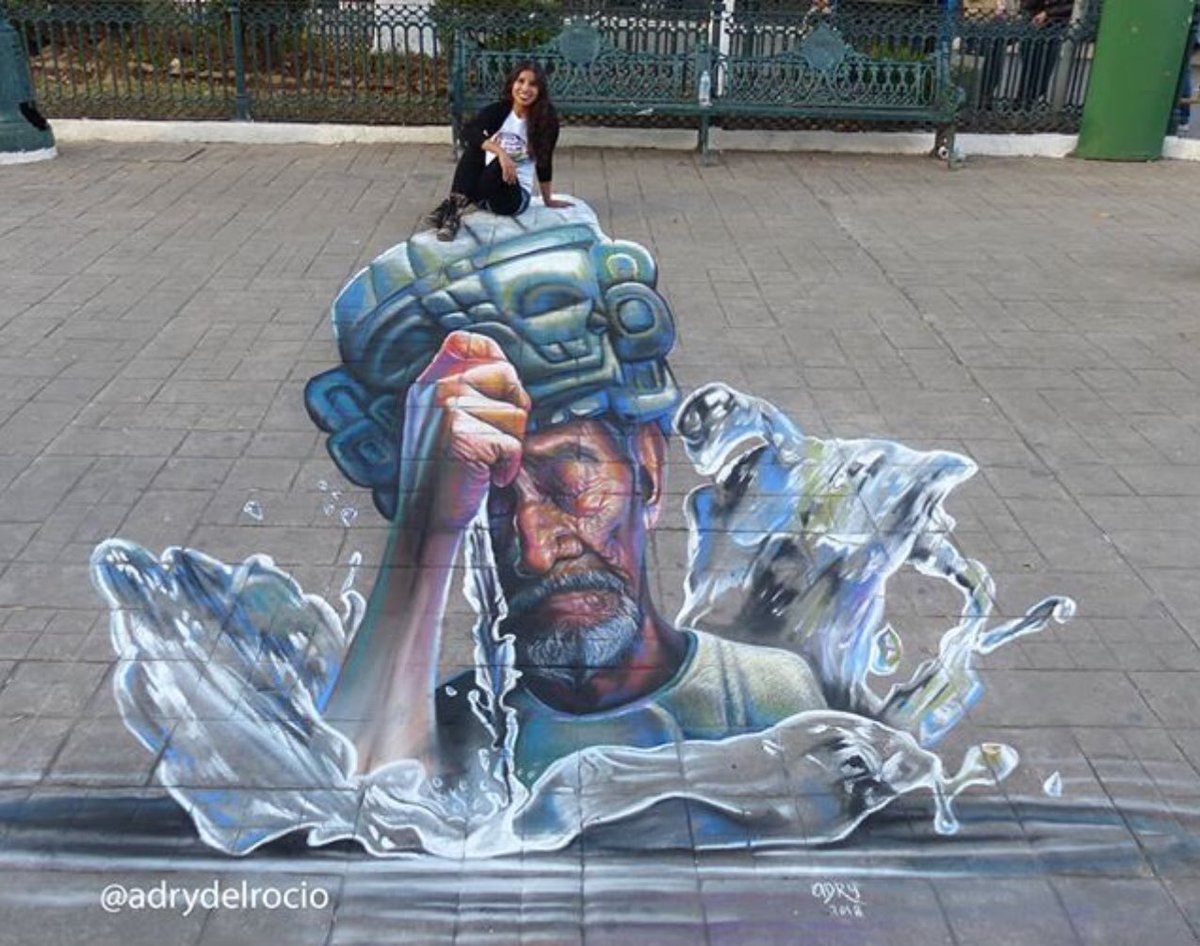The image depicts a detailed chalk mural on a reddish pavement, occupying about 90% of the frame. The mural features a brown, dark-skinned elderly man with a grey mustache and beard, his face wrinkled and eyes closed. He wears a mask on his forehead, reminiscent of a Mayan or Aztec headdress, intricately detailed in different shades of blue. His right hand is raised to his forehead, seemingly causing a splash of water to burst at the bottom, with transparent droplets highlighted in blue, green, and white. 

Sitting on top of this artistic creation is an Indian girl with long black hair, dressed in a black sweater over a white t-shirt and black leggings. She is smiling and looking directly into the camera, adding a personal touch to the scene. The background behind the pavement mural includes a metal bench, a metal fence, a patch of grass, and a green trash can in the right-hand corner. At the bottom-left corner of the mural, there's an attribution reading "ATADRY DEL ROCIO."